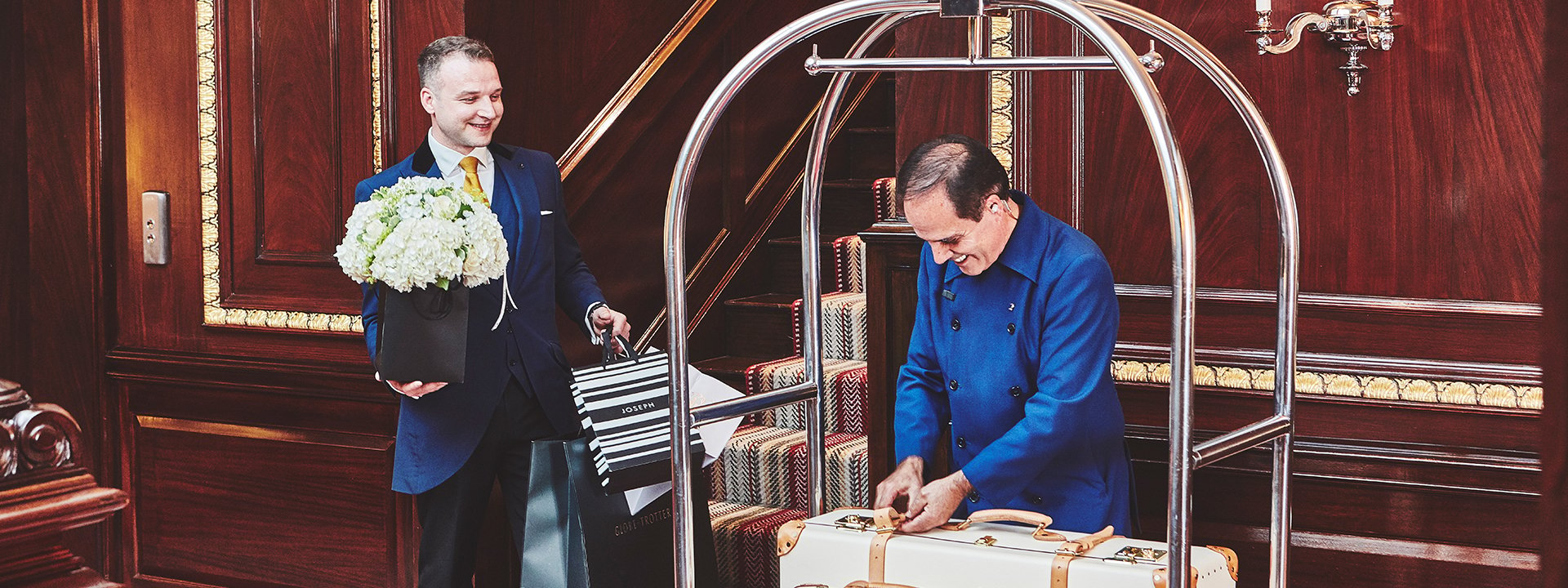The indoor photo appears to be set in an opulent hotel with a wooden interior featuring light brown accents. Central in the image is a bellhop dressed in a blue uniform, smiling as he adjusts a large white suitcase with light brown leather straps and a handle, positioned on a silver arched luggage cart. To the left of him stands a man in a blue suit jacket with dark pants and a yellow tie, holding a large bouquet of white flowers in a vase and several shopping bags in his right hand. A grand staircase ascends behind them amid the finely crafted wooden walls. The setting is further illuminated by a chandelier and additional light fixtures, adding a touch of elegance to the scene.